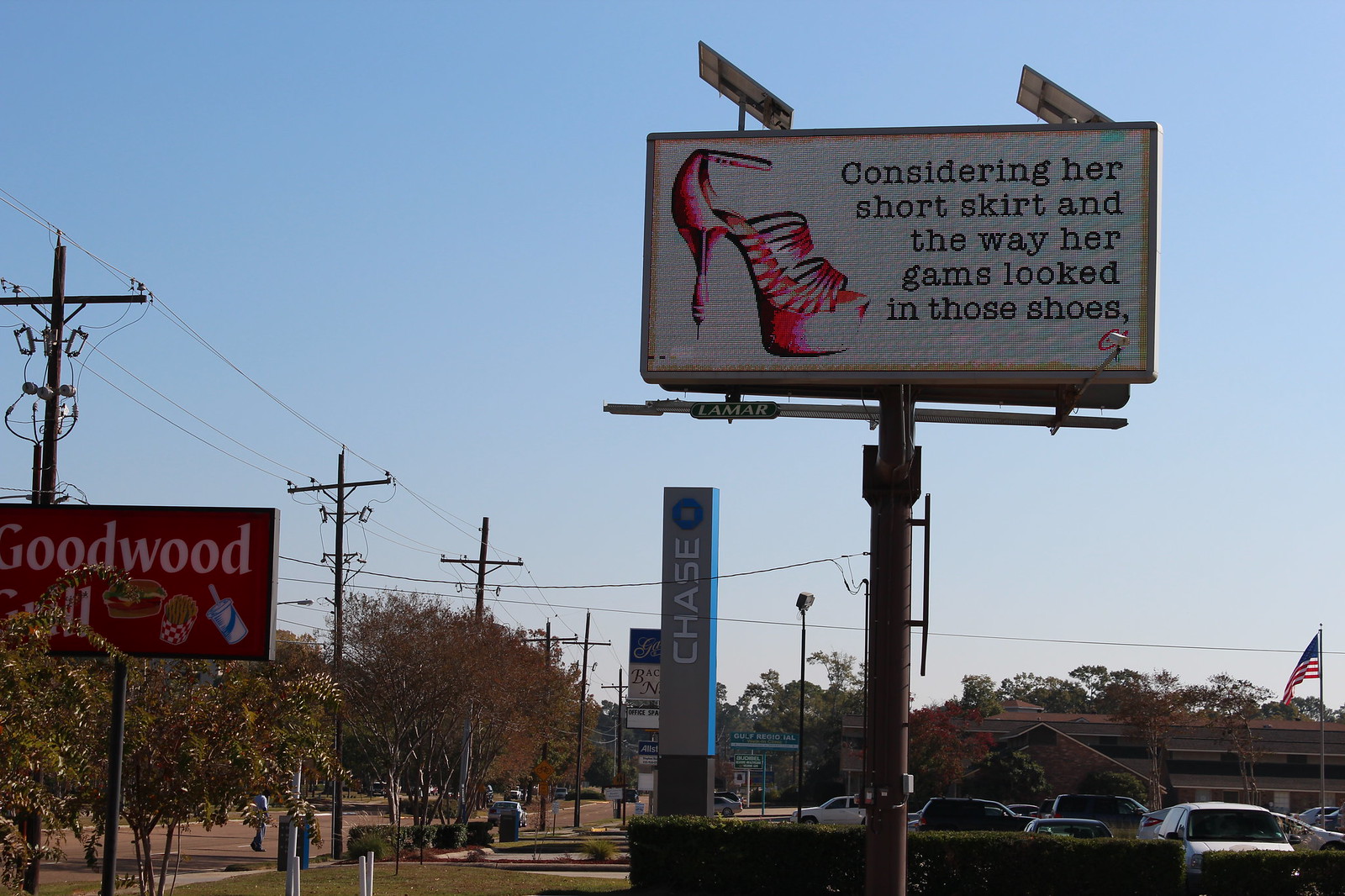The image captures a vibrant street scene centered around a towering billboard. The billboard prominently features a bright pink high-heeled shoe with a tall heel, approximately four to six inches in height, and a platform under the toe. The shoe is elaborately designed with multiple straps – one around the ankle, one across the arch, and five over the toe area. The left side of the billboard showcases this striking shoe, while the right side contains an intriguing caption written in standard font: "Considering her short skirt and the way her gams looked in those shoes." This text is set against a clean white background.

The billboard is mounted on a tall pole surrounded by well-maintained boxwood bushes. Above, the sky is blue and slightly hazy, suggesting proximity to a large city. To the left of the main billboard, a smaller sign advertises "Goodwood Grill" with an appetizing image of a burger, fries, and a drink on a red background. Below the large billboard, several electric poles are visible, along with a vertical blue sign reading "Chase."

In the foreground, there is a road accompanied by a sidewalk lined with green lawns and shorter decorative trees, contributing to the neighborhood's inviting atmosphere.